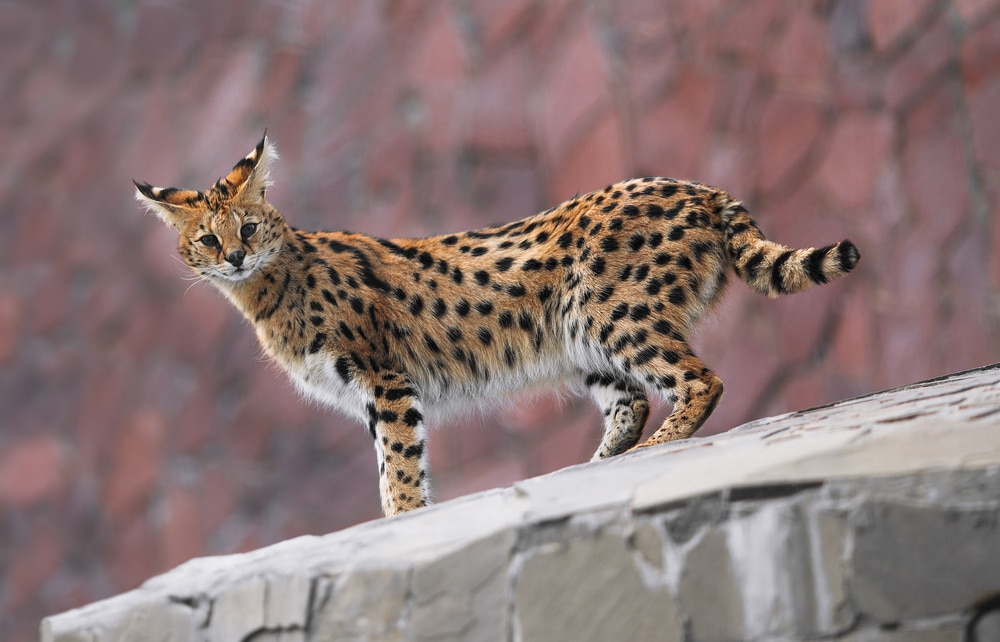The image captures a young, wild cat species, potentially a serval or a hybrid of a leopard and other wild cats, standing on a gray rock in its natural habitat. The cat's coat is orange with prominent black spots and a white trim along with noticeable stripes on its tail. It has a white belly and pointed ears with white fur on its face, which bears a closer resemblance to a domestic cat. Its long white whiskers, black nose, and brown eyes are striking features. The cat is facing the camera directly with an attentive gaze and a closed mouth. The background, slightly out of focus, consists of reddish, rusty rocks, setting a stark contrast to the gray rock the cat is perched upon.